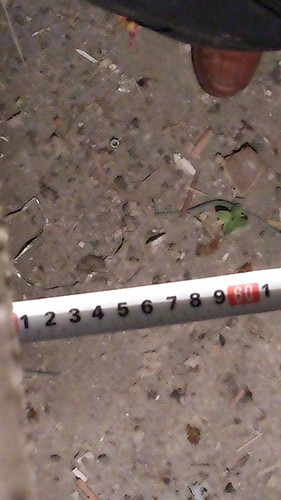The image depicts a tape measure extended on a debris-strewn surface. The tape measure shows the numbers 1 through 9, followed by a marking at 60 inches, in white letters against a red background, before resetting to the number 1. Scattered around the ruler on what appears to be a concrete or gravel surface, there are various pieces of refuse, including small fragments of wood, likely remnants from a recent windstorm. In the midst of the debris, there's a colorful green object, possibly a toy, and a solitary brown shoe positioned near the top of the image. Above the shoe, a dark area suggests a shadow or part of an object, hinting at a person possibly stepping out of a vehicle. The scene conveys a sense of disorder, with the scattered refuse and damaged objects contributing to a chaotic, post-storm atmosphere.